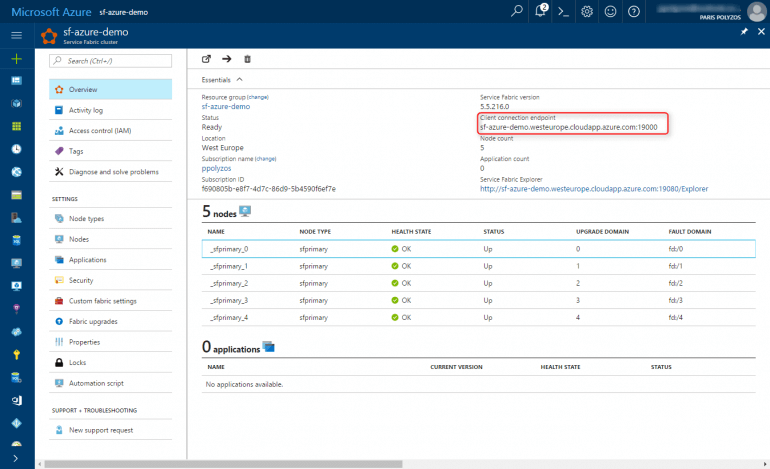This image features the user interface of Microsoft Azure. In the upper left corner, the name "Azure" is prominently displayed in light blue text. The interface's design includes a dual vertical navigation menu on the left side. The outer vertical menu, rendered in blue, seamlessly transitions into an inner vertical menu with a white background.

Further to the right, there is a highlighted red square section, delineated to capture attention. Within this section, there is information identifying a client connection endpoint labeled "AF-AZURE-demo." Below this designation, the endpoint address "westropecloud.cloudapp.azure.com" is displayed. Additionally, the number "1900" appears adjacent to this address, likely indicating a port or identifier. The image meticulously showcases the structural and navigational elements typical of Microsoft's cloud computing platform interface.